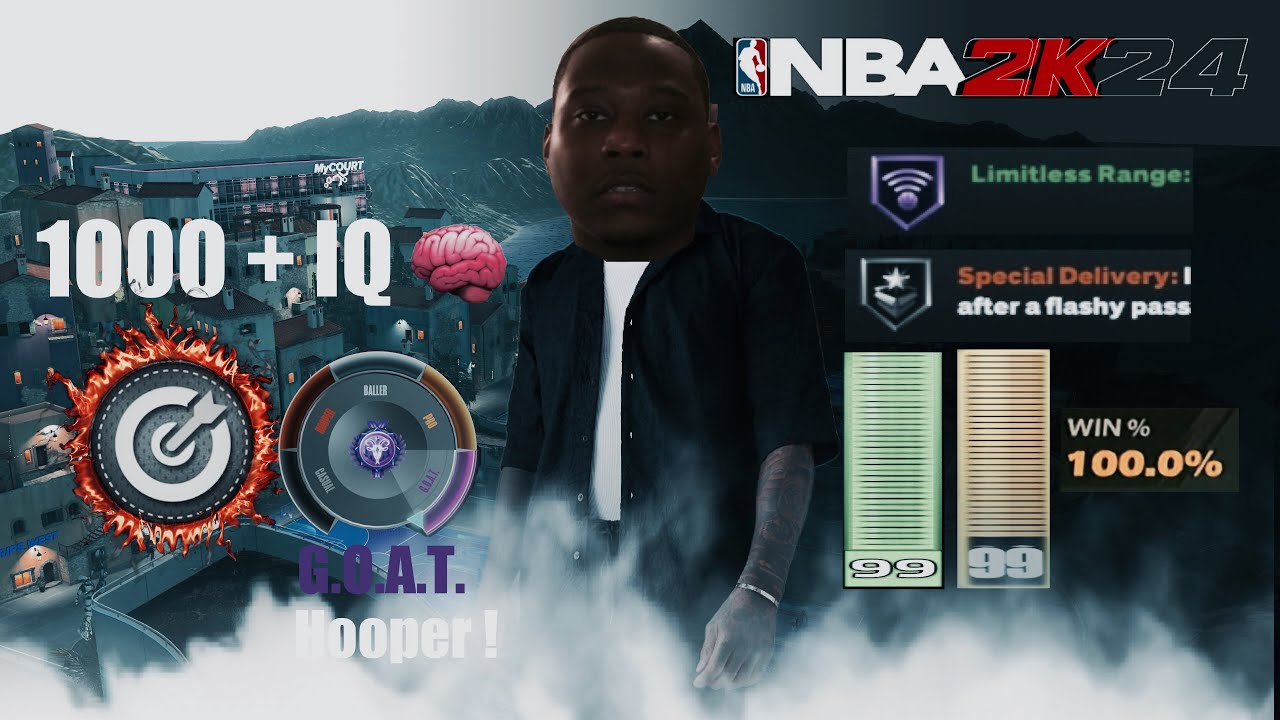This is a screenshot from the game NBA 2K24, featuring an edited meme character standing in the center of the screen, directly facing the camera. The character, a Black male with short hair, has an exaggeratedly large head and a smaller body. He is dressed in a button-up black shirt with rolled-up sleeves, left open to reveal a white shirt underneath, and his arms are tattooed. To the left of the character, text in white reads "1000+ IQ brain," accompanied by an image of a brain. Below this, there's an arrow and a target icon engulfed in flames, followed by a type of gauge. Below the icon, the acronym "GOAT" appears in purple, followed by the word "Hooper." The top right corner displays the NBA 2K24 game logo.